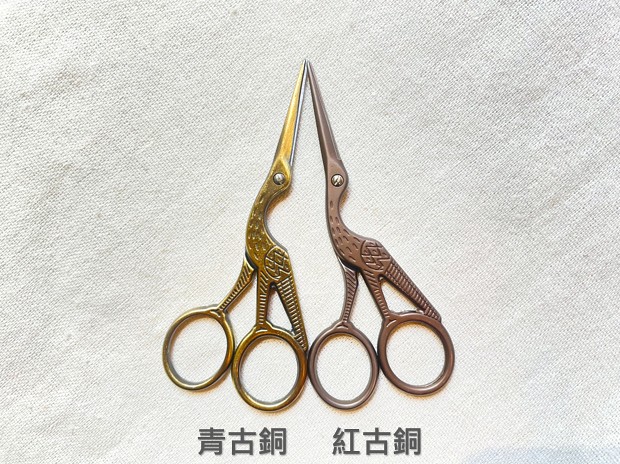The image showcases two intricately designed pairs of scissors set against a textured white fabric background. Each scissor is crafted to resemble a bird, complete with long legs, a curved neck, and a sharp beak-like blade. The left pair is made of a golden material, while the right pair is a darker metallic, possibly bronze or silver. The "eye" of each bird is represented by the screw that joins the scissor blades, and detailed engravings on the metal mimic the feathers and fur of the bird. The handles of the scissors, where fingers are inserted, form from the legs and tail of the bird, with the tail connecting to the right circular handle. Beneath each pair of scissors are several Chinese or Japanese Kanji characters, adding an oriental touch to the composition. The characters vary slightly between the two pairs, but both sets are carefully spaced under their respective scissors.